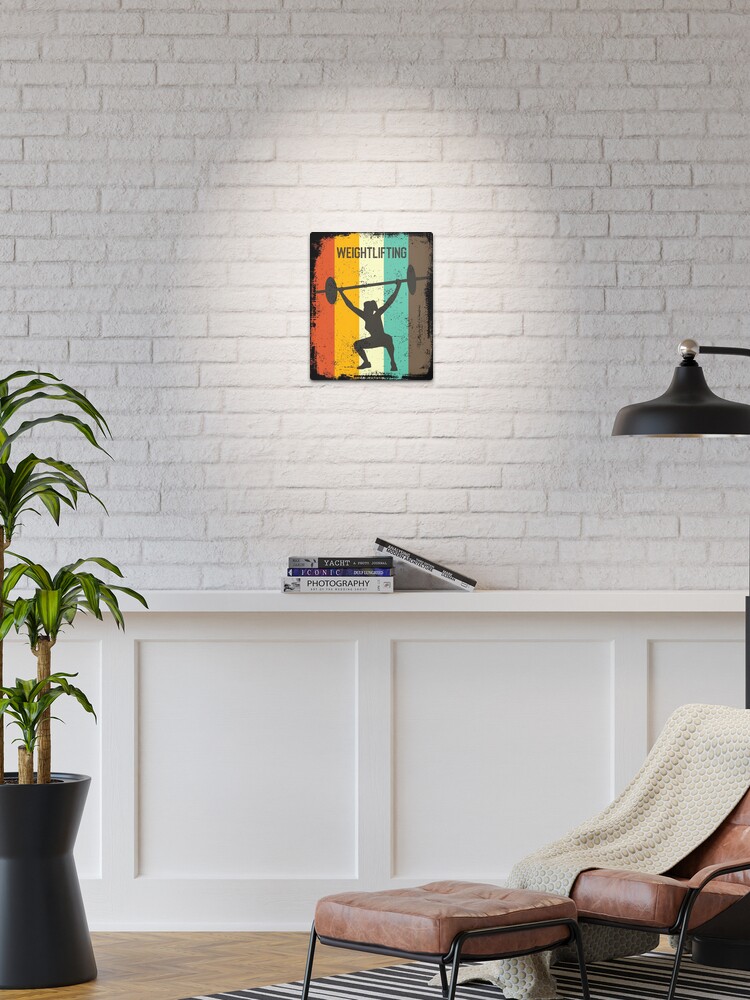The image depicts a modern, minimalist room with a stark and clean aesthetic, likely designed for a YouTube video backdrop or similar staging purpose. Dominating the background is a pure white brick wall, which creates a neutral canvas. Centrally located on the wall is a colorful picture or poster featuring the word "weightlifting" with a black image of a person lifting weights against vibrant stripes in pink, orange, yellow, green, and brown.

Below the picture is a white shelf holding five staged books, one of which has "photography" written on the spine. To the left of this shelf stands a tall plant in a black planter, adding a touch of greenery to the otherwise monochromatic setting.

On the right side of the image is a sleek, modern brown leather chair with black metal trim, accompanied by a matching brown footstool. Draped over the chair is a beige or white throw blanket, lending a cozy touch. Above the chair, a black lamp is turned on, casting light onto the white brick wall. The flooring appears to be wooden, partially covered by a black and white striped throw rug. The overall atmosphere is minimalist, with a limited color palette that emphasizes the colorful poster on the wall. This setup could either be for a home preview or a neatly arranged bachelor pad.